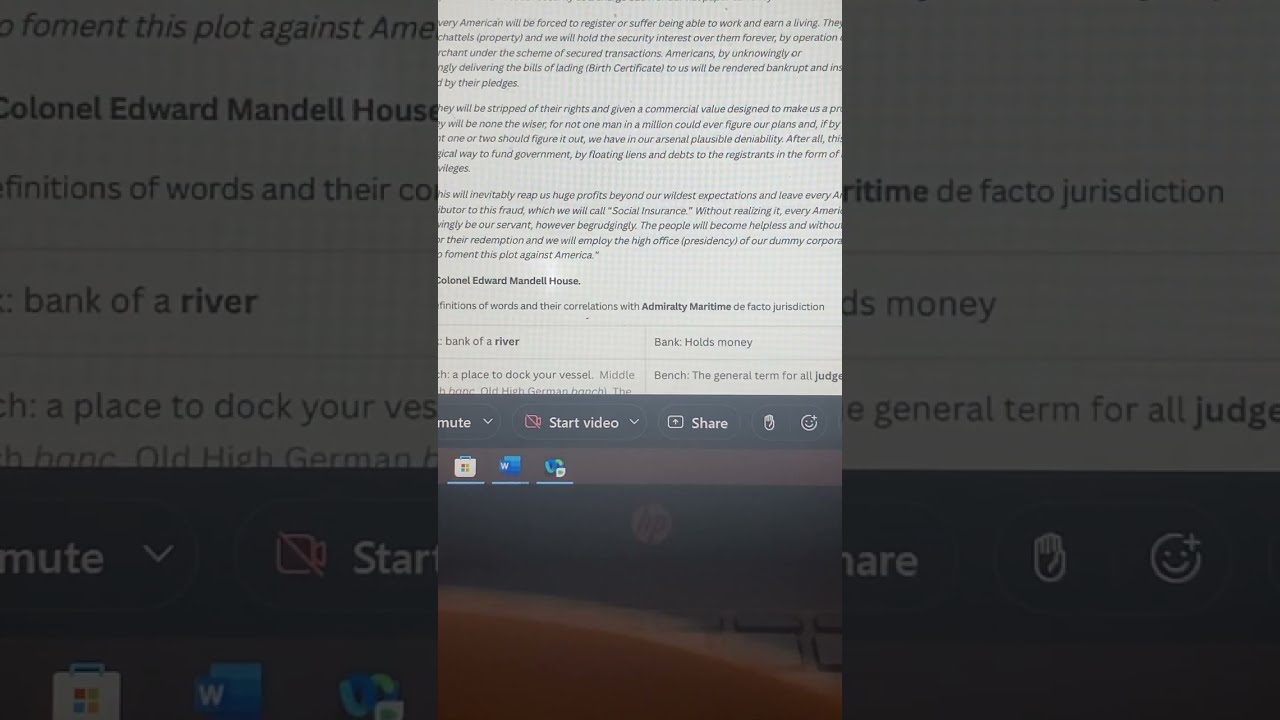The image is a screenshot of a computer monitor displayed in a vertical orientation. The central portion of the screenshot showcases a lighter section of the screen containing a white background with several paragraphs of black text, resembling a test or a document. Positioned below this text are buttons and icons, including "start video" and "share," each accompanied by small icons—a camera for starting a video. The taskbar at the bottom features additional icons such as the Microsoft Edge or Safari icon, Microsoft Word symbol, and the App Store symbol.

On both the left and right sides of the central image are darker, more zoomed-in sections that show close-ups of parts of the text featured in the central area. These side sections are somewhat blurry and darkened, creating a contrast with the clearer lightened center. Alongside the start and share buttons, other notable elements including the mute button, a hand icon, and a smiley face emoji symbol are visible. Specific phrases like "Bank of River," "Colonel Edward Mandel House," and "a general term for all judges" are discernible within these various sections of text.